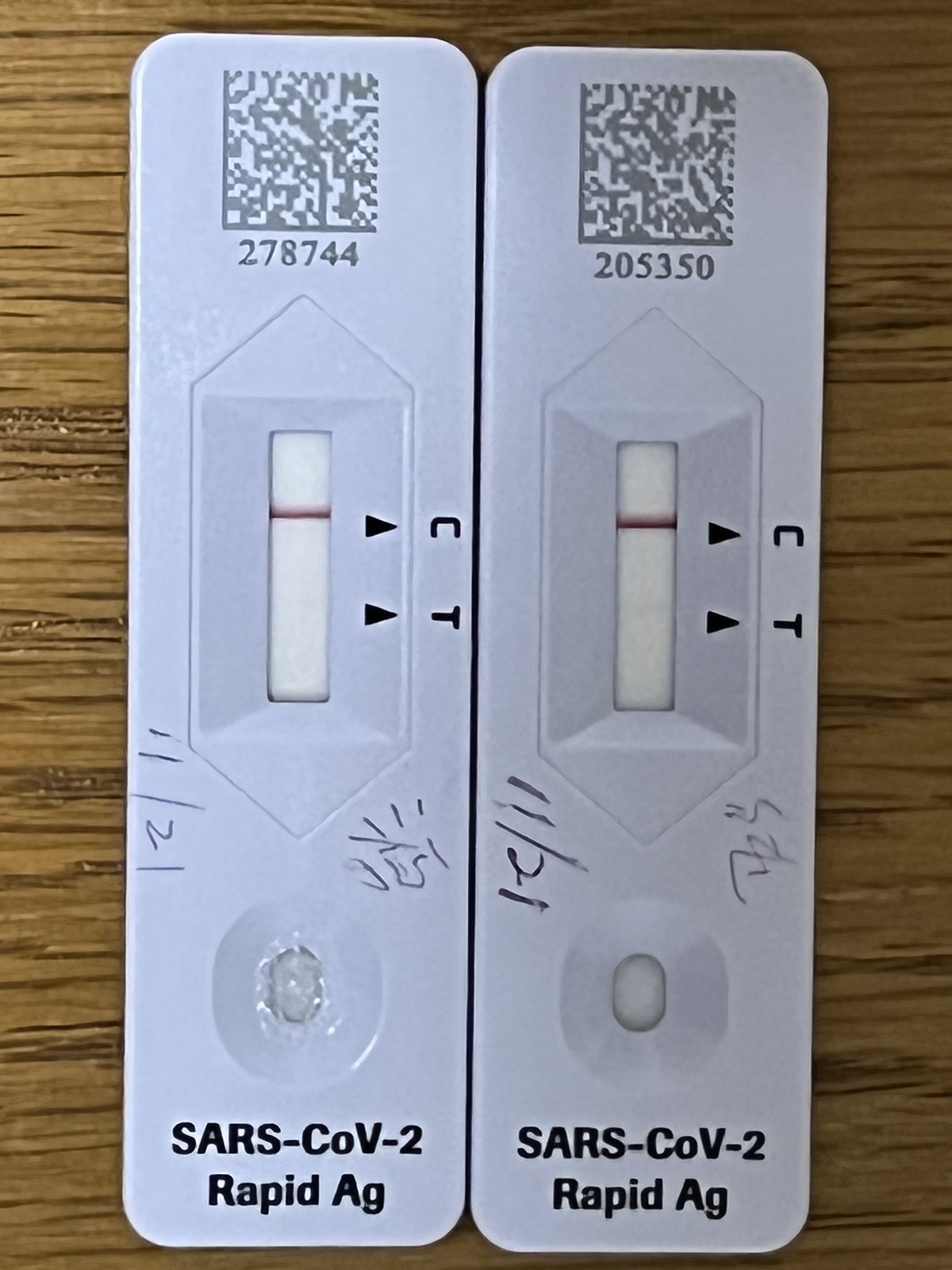The image presents two COVID-19 rapid antigen tests placed side-by-side, oriented vertically on a brown woodgrain table. Each test is marked with a unique identifier—278744 on the left and 205350 on the right—positioned beneath a QR code. Both tests showcase a vertical rectangular window with a dark horizontal line aligned with the 'C' marker, indicating the control line. There is an arrow pointing to the 'T' marker in each window, but no visible lines are present at this level, suggesting a negative result for each test. The background within these windows is white. Along the side of both tests, the numbers "11/21" are displayed, presumably indicating the date of manufacture or expiration. At the bottom of these tests, a circular indentation is present, and directly beneath it, the label "SARS-COV-2 Rapid A-G" is printed.